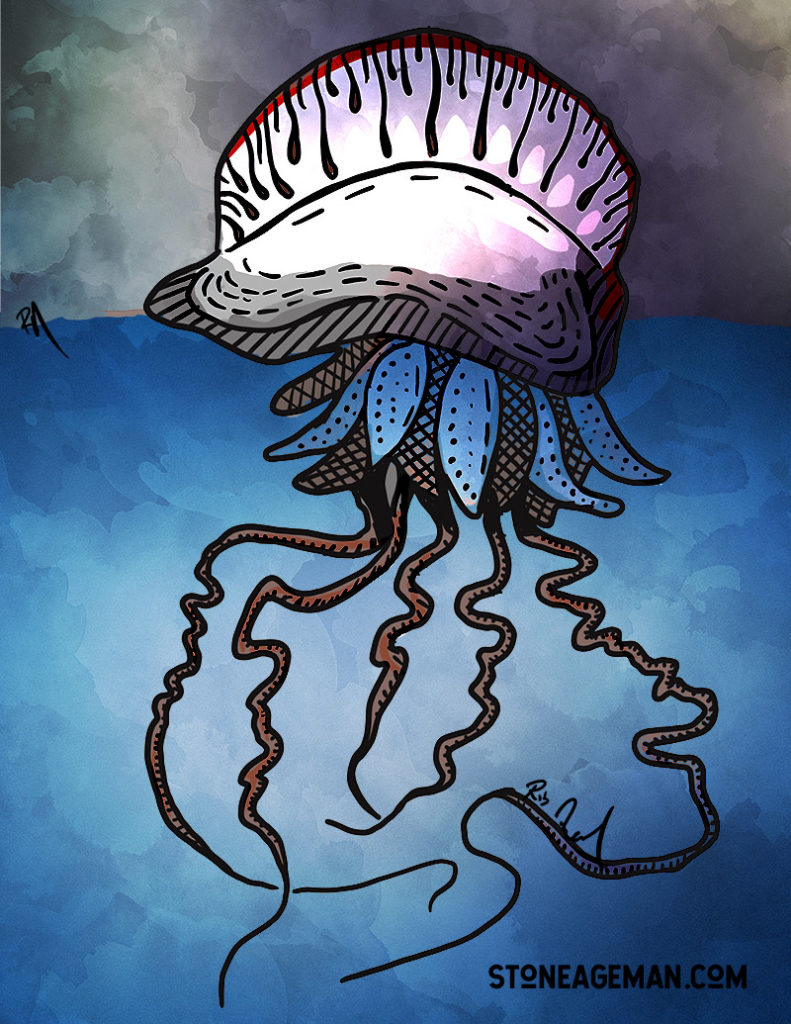This artwork, likely a modern watercolor painting, features an abstract and vibrant depiction of a marine creature, resembling an octopus or jellyfish, set against a dramatic gray stormy sky and deep blue waters. The creature's body, highlighted in tones of black, white, gray, and red, shows dual traits resembling tentacles and squiggles, extending in light brown hues. Its upper body, evocative of a jellyfish dome, displays a clear form with vertical stripes and a distinctive red band. A subtle blue leaf-like structure adds to its ethereal quality. The bottom of the image prominently features the signature "StoneAgeMan.com" in black text, further emphasizing the artist's modern and abstract style.